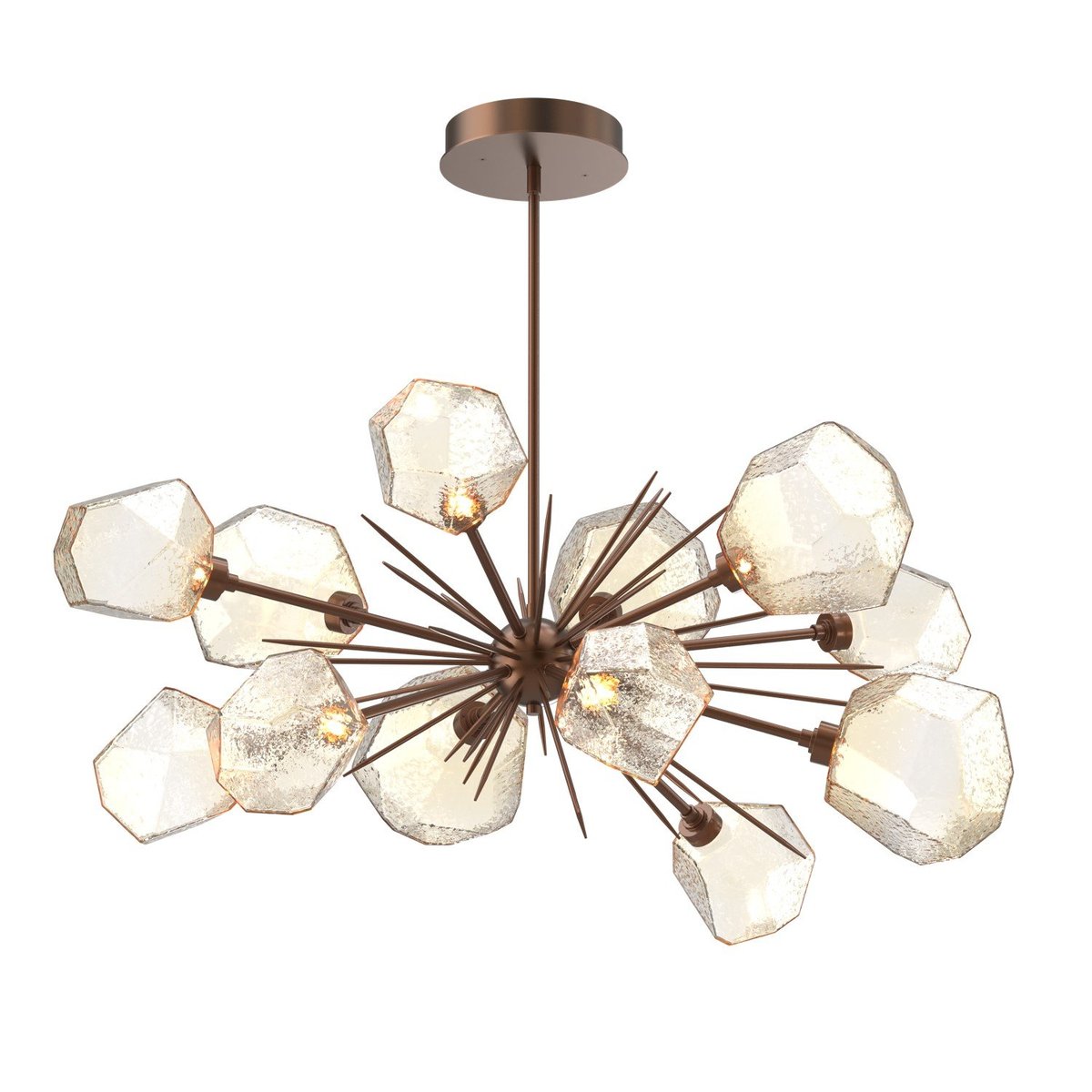This color photograph captures a modern, pendant-style chandelier suspended against a white background, giving the impression that it is floating. The chandelier is anchored to the ceiling by a round, brass-colored mount, from which a vertical, brown rod descends. This rod connects to a central spherical hub made of the same brassy copper material. From this central sphere, an array of spiky, brown rods radiates in all directions, resembling the stems of a flower. These rods vary in length, and some culminate in unique, jagged, angular light bulbs that resemble chunks of ice. The twelve off-white, faceted glass bulbs, each with a pentagonal or square-like shape and petal-like sections, contribute to the chandelier’s modern aesthetic. This detailed image is reminiscent of product photography typically seen on shopping websites like Home Depot, emphasizing the fixture’s intricate design and contemporary style.